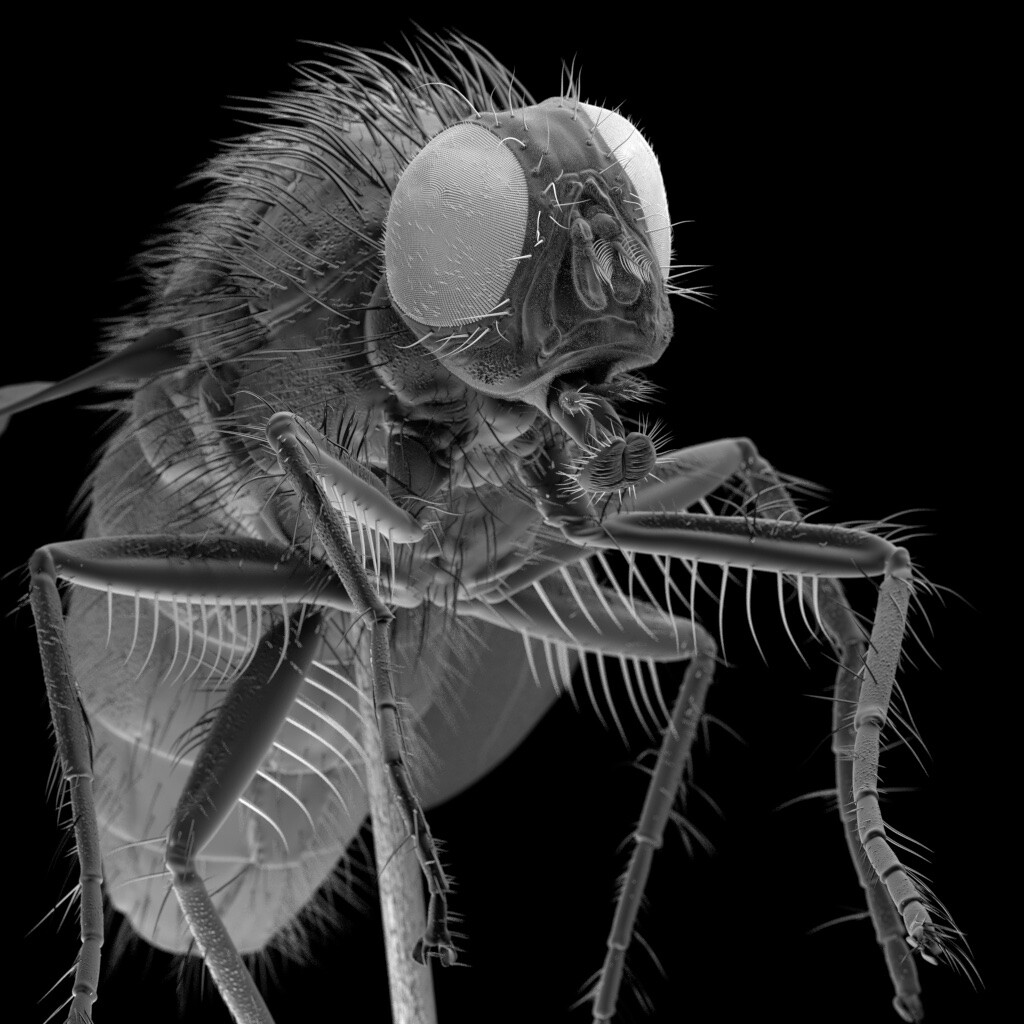This monochromatic image depicts a highly detailed, 3D drawing of a fly positioned against a black background. The perspective offers a front view of the insect, showcasing its two large, mesh-covered eyes and an open mouth. The insect's body, rendered primarily in shades of grey, features an elongated backside and a set of six legs adorned with numerous fine, hair-like structures. These fibrous details are also present on the fly's body, emphasizing the intricate textures. The head of the fly is centered in the image, while its body trails behind and to the left. This high-definition image, which resembles a microscopic view, captures the nuanced features of the fly with impressive clarity.